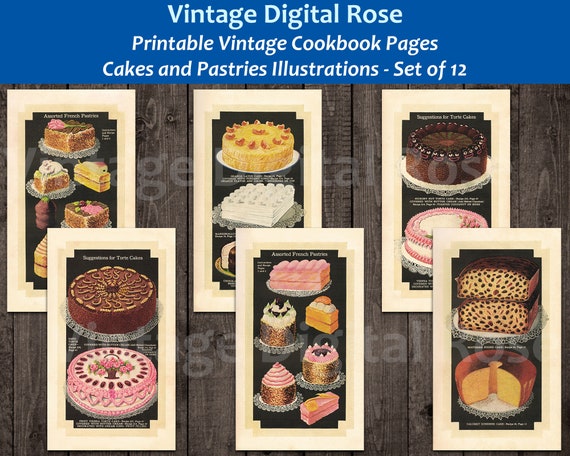The image showcases a detailed digital illustration of vintage cookbook pages, specifically focusing on cakes and pastries. It features six rectangular illustrations divided into two rows, with three in the front and three partially hidden behind them. Each illustration highlights different types of cakes, including individual-sized cakes, bundt cakes, and what appear to be strawberry and chocolate cakes. The illustrations are arranged over a wooden background. At the top of the image, a blue horizontal banner contains the text "Vintage Digital Rose, Printable Vintage Cookbook Pages, Cakes and Pastries Illustrations - Set of 12," emphasizing the collection and its vintage aesthetic. Additionally, a translucent white overlay repeats the title "Vintage Digital Rose" across the sets.